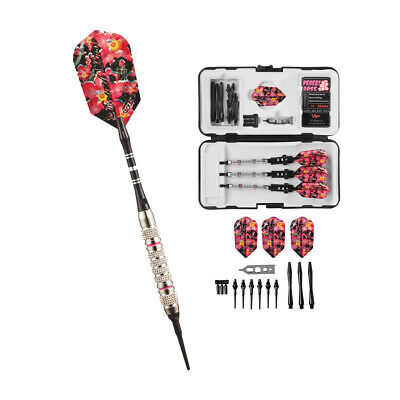The image is a professionally shot product photograph of a dart set, designed for commercial use in online shops, listings, or catalogs. The photograph is rectangular with a featureless white background, creating the illusion that the dart set is floating. The main focus is an ornate, fully assembled dart on the left side of the photograph. This dart features a finely pointed black plastic needle at the front, followed by a metallic silver ridged handle with two red stripes, and a black rod. The dart is adorned with pink and black floral-designed fins at the rear, adding a striking visual element.

To the right of the assembled dart is an open black case with a white foam interior, showcasing three identical darts neatly lined up in the bottom half. The top half of the case holds spare tips and flights. Below the case, individual components are meticulously displayed, including three flights with a floral design, additional pointed tips, and other essential parts of the dart set. This detailed arrangement highlights the comprehensive nature of the kit, making it clear what the package contains.